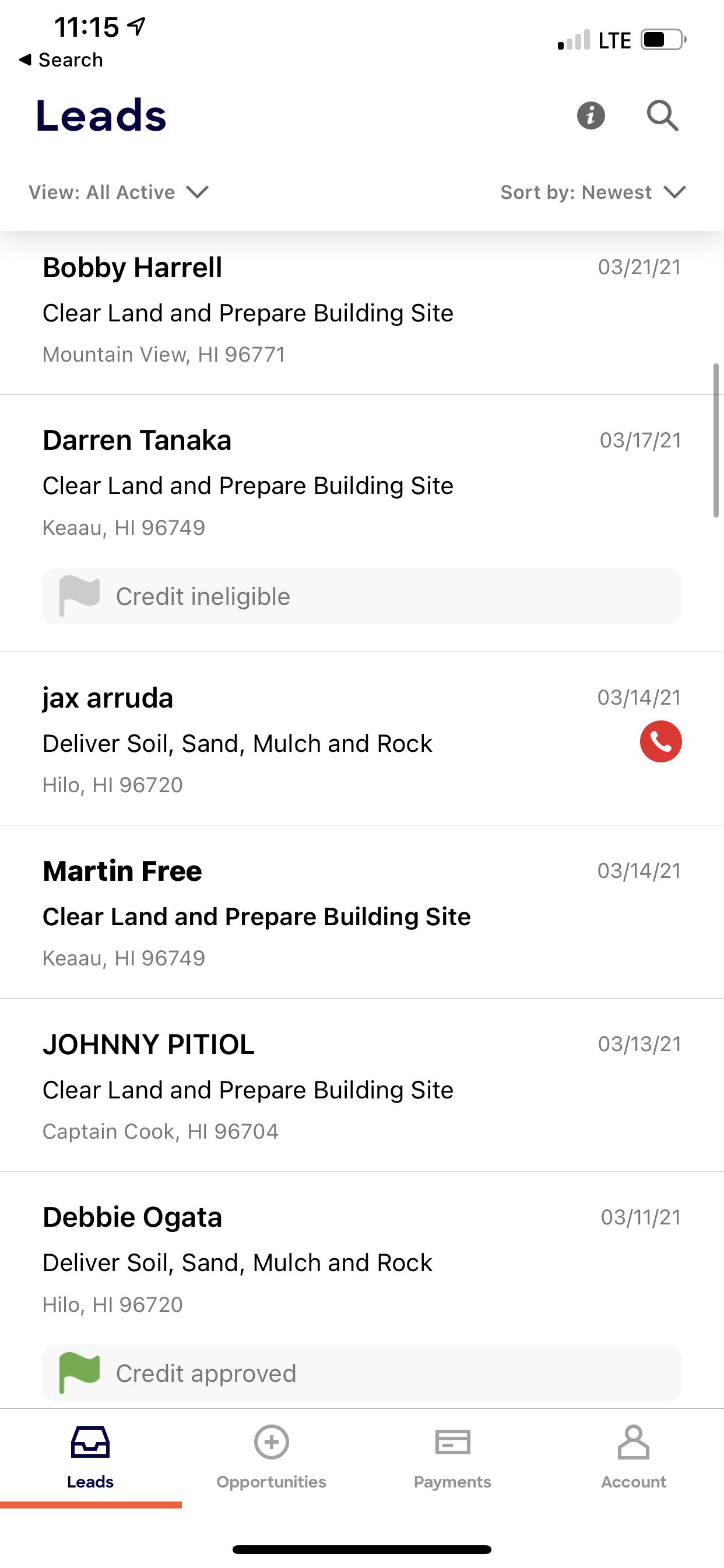Screenshot of a cell phone screen featuring a white background with black text. At the top of the screen, "11:15" is displayed next to a GPS icon. On the right-hand side, it shows 1 out of 4 bars for signal strength, "LTE," and a half-full battery icon.

Beneath the time display on the left, there is a back arrow followed by the word "Search." Underneath, "Leads" is prominently displayed. On the right, gray icons include a circle with a slash through it and a magnifying glass. Below this, there's a gray bar that reads "View All Active" with a down arrow next to it and "Sort by Newest" with another down arrow on the right side.

The main section of the screenshot lists multiple leads. On the left side, dates are shown in gray text, and the corresponding information is in black on the right:

1. **Bobby Harrell:** Clear land and prepare building site, dated 03-21-21.
2. **Darren Tontaka:** Clear land and prepare building site, dated 01-17-21. Note: credit details are illegible.
3. **Jacks Aurora:** Deliver soil, sand, mulch, and rock, dated 03-14-21. A phone icon suggests this person can be contacted directly.
4. **Martin Free:** Clear land and prepare building site, dated 01-13-21.
5. **Jonathan Pittle:** Clear land and prepare building site, dated 01-13-21.
6. **Debbie Ortega:** Deliver soil, mulch, and rock, dated 01-11-21. Note: her credit is approved.

The location of these leads is noted to be in Hawaii. At the bottom of the screen, menu options include "Leads," "Opportunities," "Payments," and "Account."